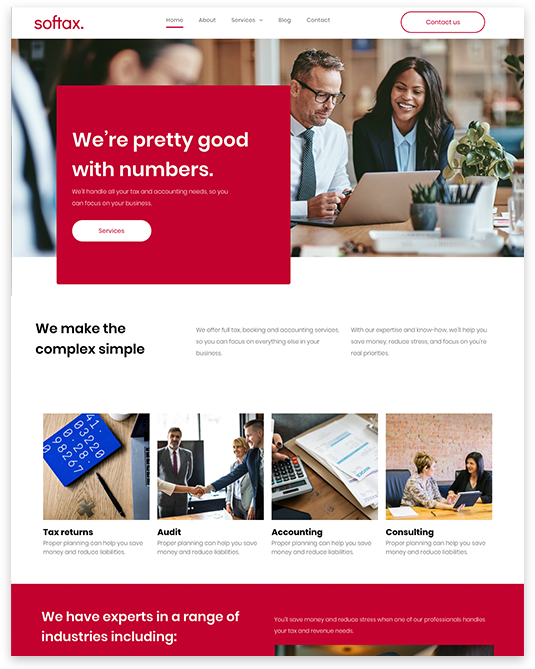This image is an advertisement photo for the Softax website, showcasing the partially visible front page. The top part of the website is depicted, with the bottom half cut off. In the upper left corner, the Softax logo is displayed prominently. To the right of the logo, five categories are centered at the top of the page, with the "Home" category selected and highlighted by an underscored red bar. 

In the far right corner, a "Contact Us" button is prominent. Below the header, the background features a photo of individuals gathered in a boardroom around a computer, suggesting collaboration and professionalism. Overlaid on the left side of this photo is a red text box with the bold white statement, "We're pretty good with numbers," accompanied by a white "Services" button beneath it.

The page transitions to a white background below the photo. At the lower section of the image, there is a row of thumbnails representing different categories such as "Audit," "Accounting," and "Consulting." At the very bottom of the page, partially cropped out on the right side is another red box containing the top portion of an additional photo.